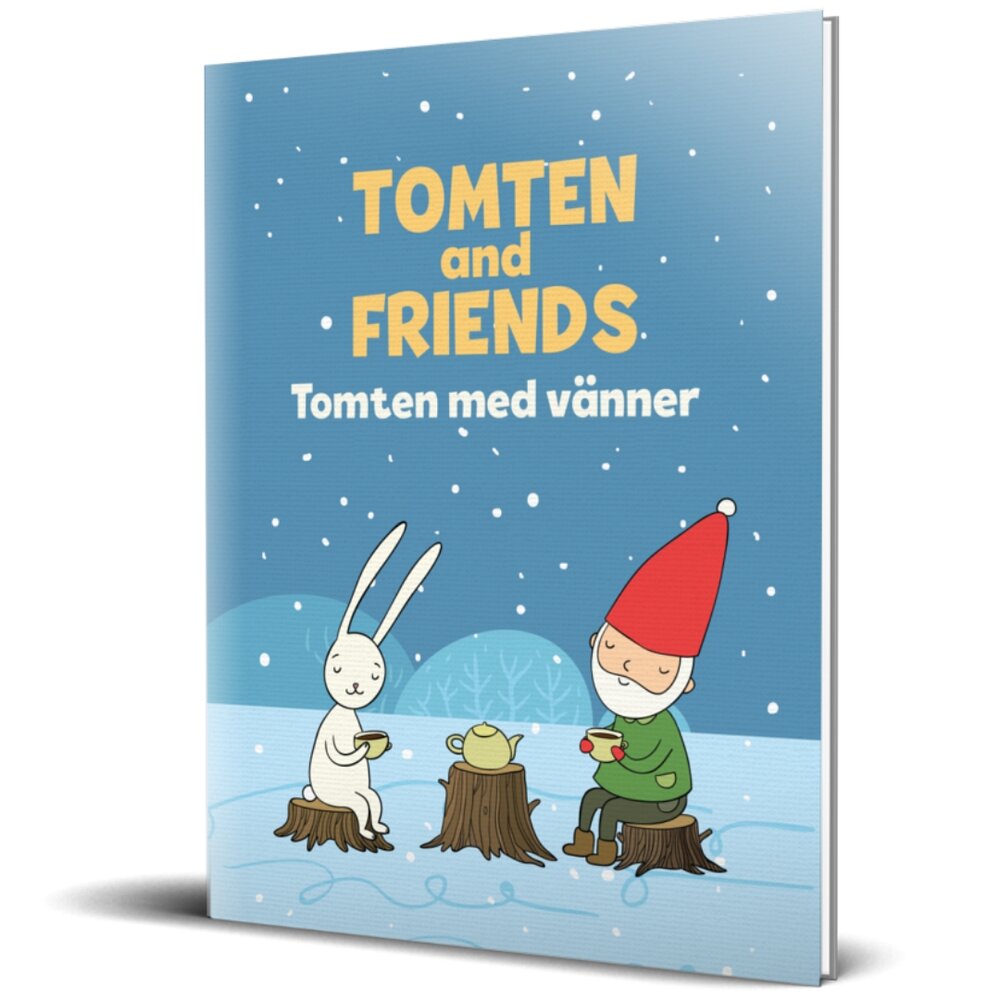The cover of the picture book titled "Tomten and Friends" (Tomten Med Vänner), set in a snowy landscape with falling snow and trees in the background, features a cozy, heartwarming scene. On the left, a bunny with white fur sits on a tree stump, eyes closed, savoring a cup of steaming tea or coffee. To the right, a gnome or elf figure, distinguished by a long red hat, a green shirt, red mittens, black pants, brown boots, and a white beard, also sits on a stump, mirroring the bunny's peaceful posture while enjoying a similar warm beverage. Positioned between them is a larger tree stump serving as a table, holding a matching green teapot. The entire scene is depicted in a charming cartoon style, emphasizing the tranquil camaraderie on this snowy day. The blue-hued background, accentuating the serene winter atmosphere, contrasts vividly with the colorful characters and objects.